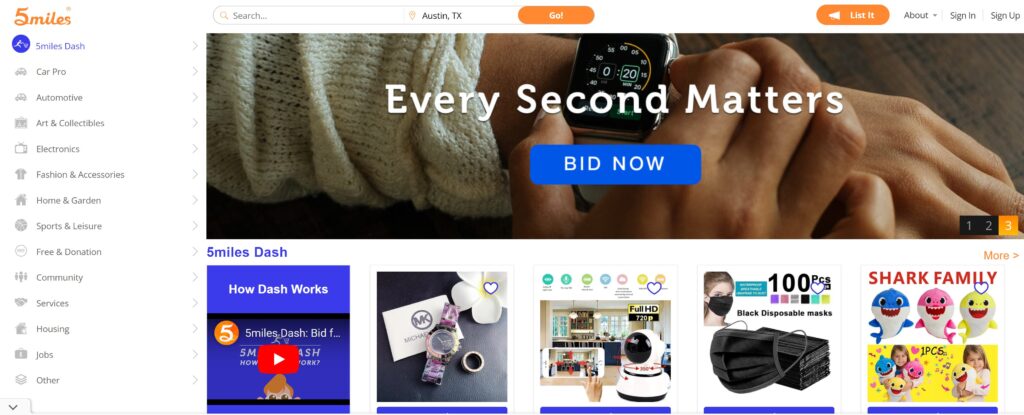Screenshot of a vibrant web page featuring a large banner at the top. The banner displays a photo of a pair of hands, conveying a sense of urgency with the bold text "Every Second Matters." Below the text is a prominent call-to-action button reading "Bid Now." Scrolling down, we encounter a row of five distinct images. 

The first image is a screenshot of a video, highlighted with a purple overlay that reads "How Dash Works." 

The second image showcases a pink watch elegantly placed next to a white jewelry dish atop a white card, exuding a sense of style and simplicity.

Next, the third image captures an automatic litter box, available in multiple colors, depicted against the backdrop of a cozy home interior.

The fourth image presents a stack of 100 black COVID masks, accompanied by an inset of a woman wearing one, emphasizing both the quantity and practical use of the product.

Finally, the fifth image features three different toy sharks, labeled "Shark Family." Below this, a yellow box frames two little girls, each playfully holding one of these shark toys, adding a touch of charm and relatability to the scene.